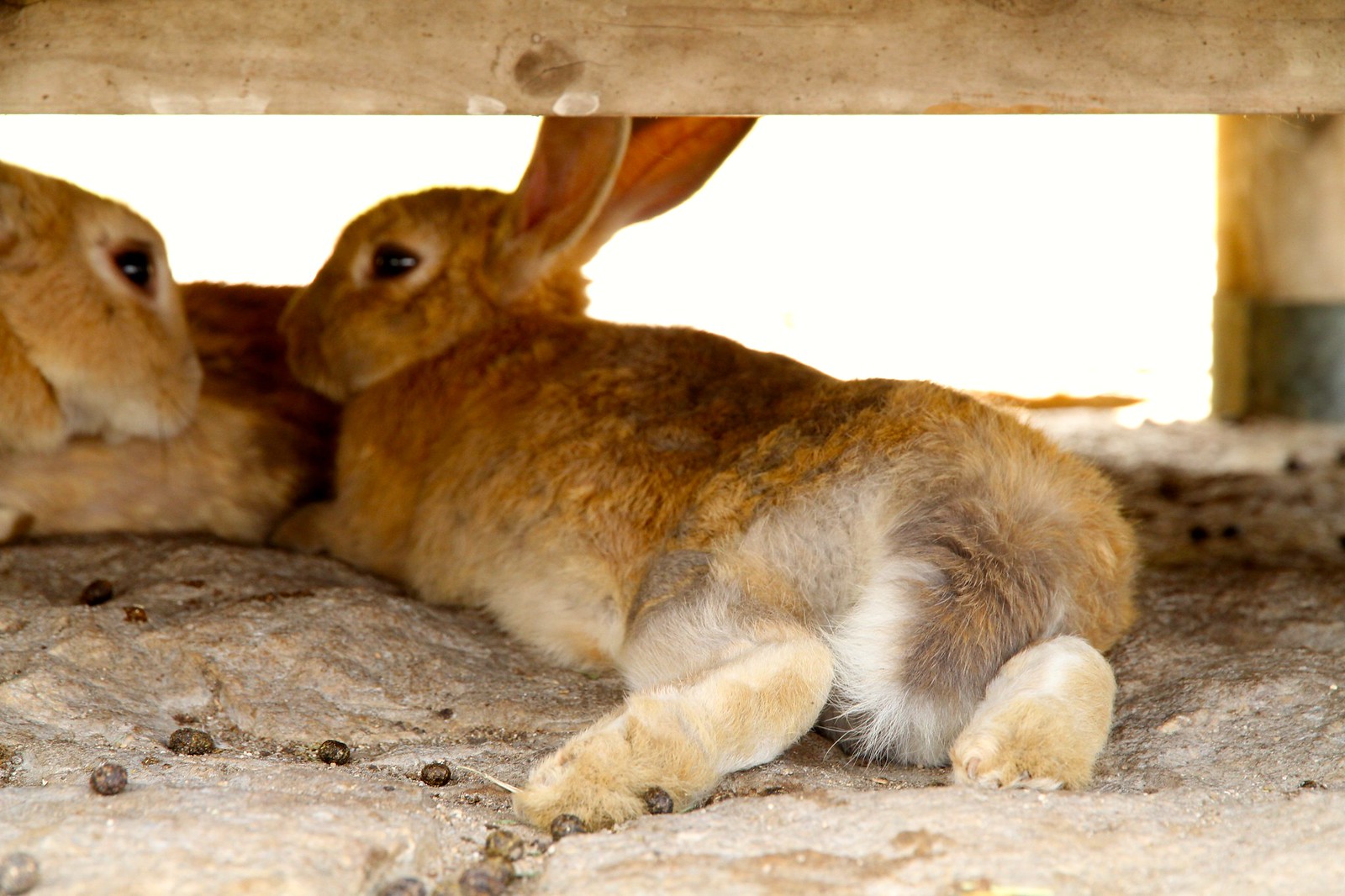This photograph captures two adorable bunnies relaxing in what appears to be a wooden rabbit hutch. The hutch, constructed from brown wood, provides a cozy den-like setting for these rabbits, which have a distinctive reddish-golden, almost orange fur. The ground of the hutch is scattered with small, brown rabbit droppings, which are visible throughout the image.

The central bunny, positioned prominently, is stretched out with its rear end closest to the viewer, facing slightly to the left. Its ears are perked up, and its body extends out with an alert yet relaxed posture. This bunny’s coat is a striking orange-gold color, and although its feet appear a bit dirty, likely from the hutch’s conditions, it still maintains a clean look overall.

To the left side of the image, the second bunny’s head peeks out, its body mostly hidden. This bunny is also looking to the right, showcasing its soft fur and creating a charming scene of curiosity and relaxation.

The floor of the hutch might be made of a solid, possibly rocky material, which adds to the rustic charm of their home. Soft light illuminates the setting, highlighting the bunnies' fluffy tails and further adding to the adorable appeal of the scene.